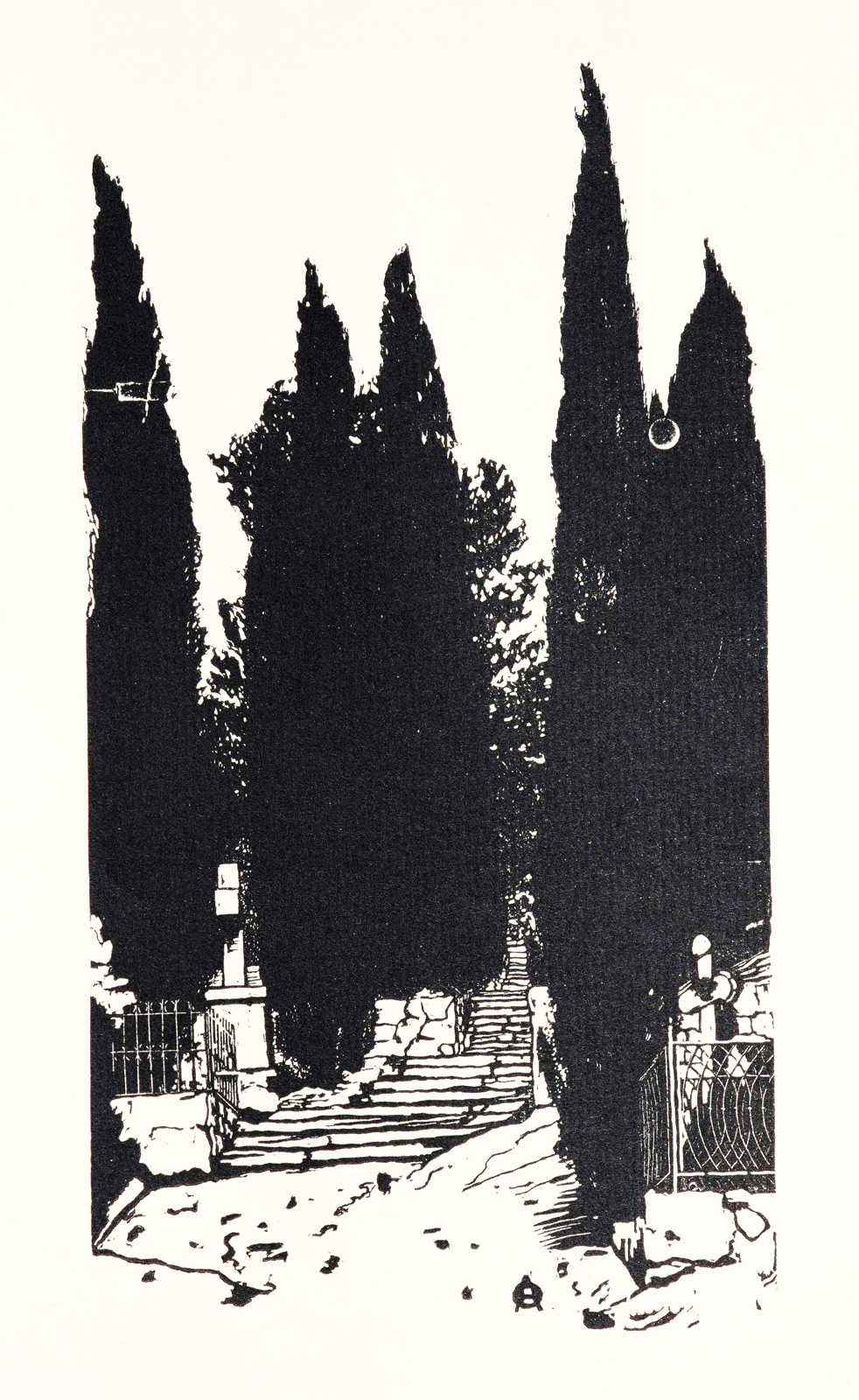This is a vertically oriented, black and white illustration on slightly aged white paper, featuring a landscape with tall, spindly pine trees. There are five prominent evergreens in the foreground; their tips reach towards the upper portion of the image. Behind these trees is another large tree with branches and leaves.

The scene appears to be set in a garden or cemetery. In the foreground, a staircase made of white slats with black outlines ascends into the distance, flanked on either side by wrought iron fencing. On the left of the stairs, there's a tombstone adorned with a cross, further suggesting a cemetery setting. The stairs lead through the trees to an indistinct terminus, creating a haunting and serene atmosphere. No figures are present in the image, and there are no borders or clouds depicted against the very light pink background.